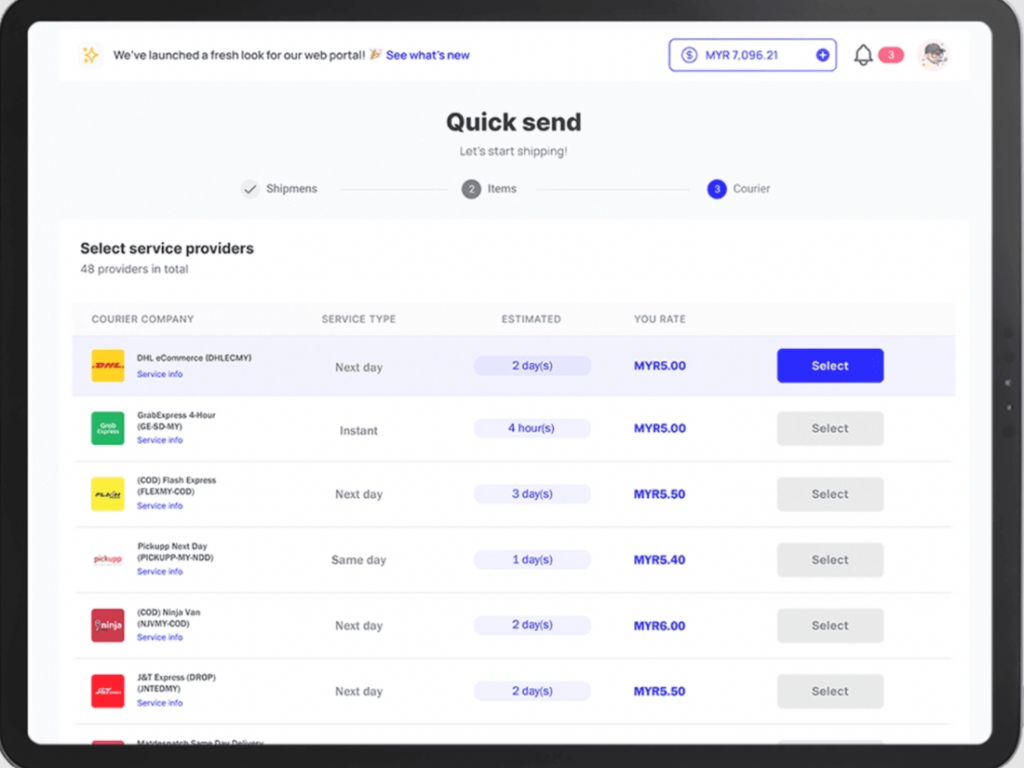Screenshot of a tablet showcasing a newly redesigned web portal. 

In the upper left-hand corner, a star emoji introduces an announcement: "We've launched a fresh look for our web portal. See what's new." Moving to the upper right-hand corner, the text displays "MYR7,096.21," next to a bell emoji indicating three notifications. 

The user's avatar appears to be a self-drawn image. The main content of the screen focuses on a feature titled "Quick Send: Let's Start Shipping," listing three main criteria: "Shipments" with a check mark, "Two Items," and "Three Couriers."

Below this main message, the section titled "Select Service Providers" reveals details with 48 providers listed in categories such as courier company, service type, estimated delivery time, and rate. The user has selected DHL eCommerce for next day service with an estimated two-day shipping time, costing MYR 5.00.

The background of the portal is white, and it displays numerous other courier options, all promising delivery times ranging from one to three days and offering similar pricing.